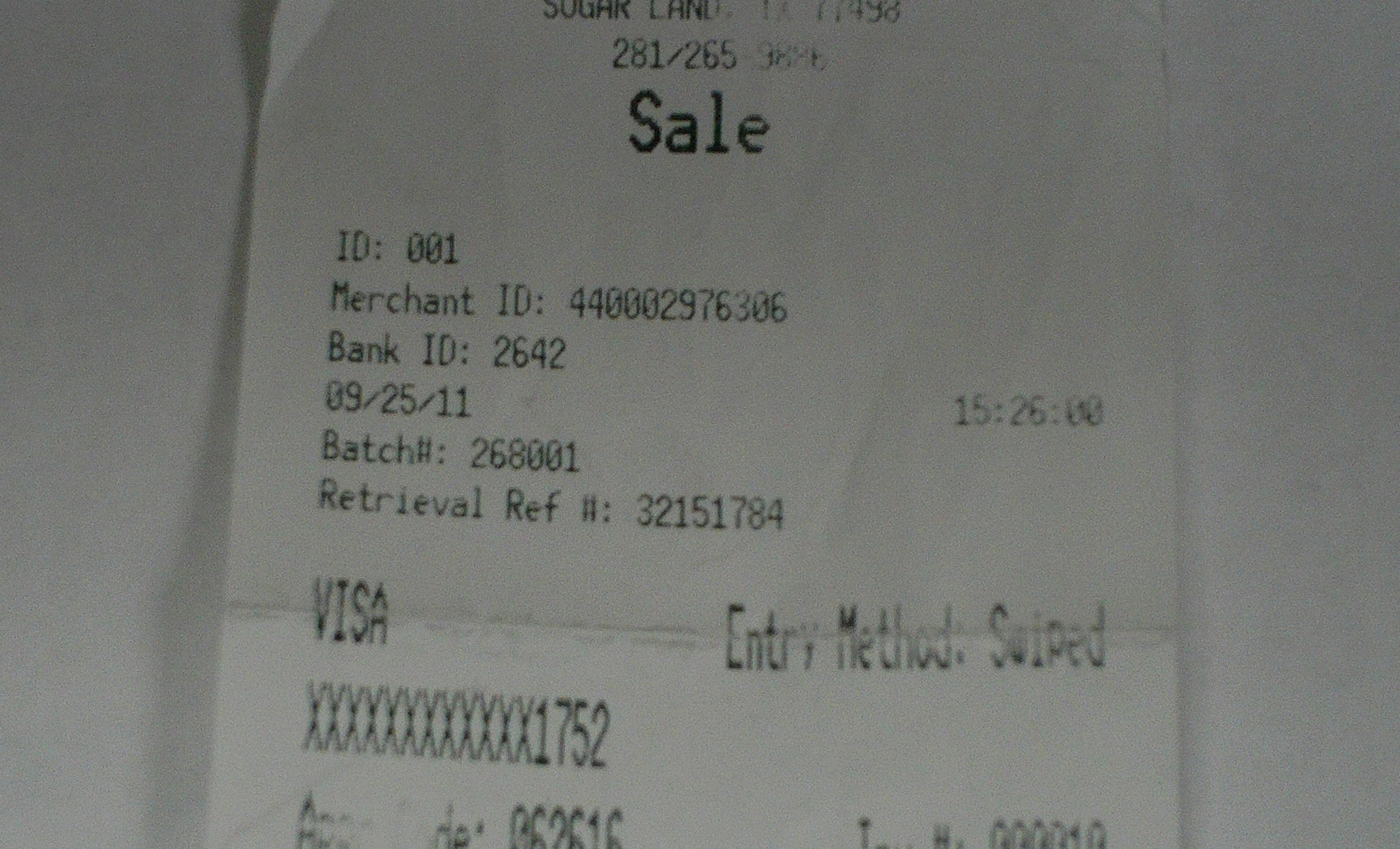This detailed photograph captures an up-close image of a white receipt lying on a white background. At the top of the receipt, the partially readable business name might include the word "Sugar". Just below this, there are various identifiers: sale number 281-265 prominently displayed, followed by "SELL" in large black letters, and an ID labeled as 001. Further down, the merchant ID features a large number, alongside a bank ID numbered 2642.

The receipt is dated 09-25-11 and indicates a batch number #268001. The retrieval reference number is provided as 321-51784. In clear capital letters, the receipt states that the payment was made using a VISA card, with the entry method listed as 'swipe'. Near the VISA indication, the receipt shows a series of Xs concealing part of the card number, revealing only the last four digits: 1752. The text on the receipt appears black and legible, though some content at the bottom is cut off, likely due to the image cropping. The receipt also seems to have visible creases, suggesting it has been folded.